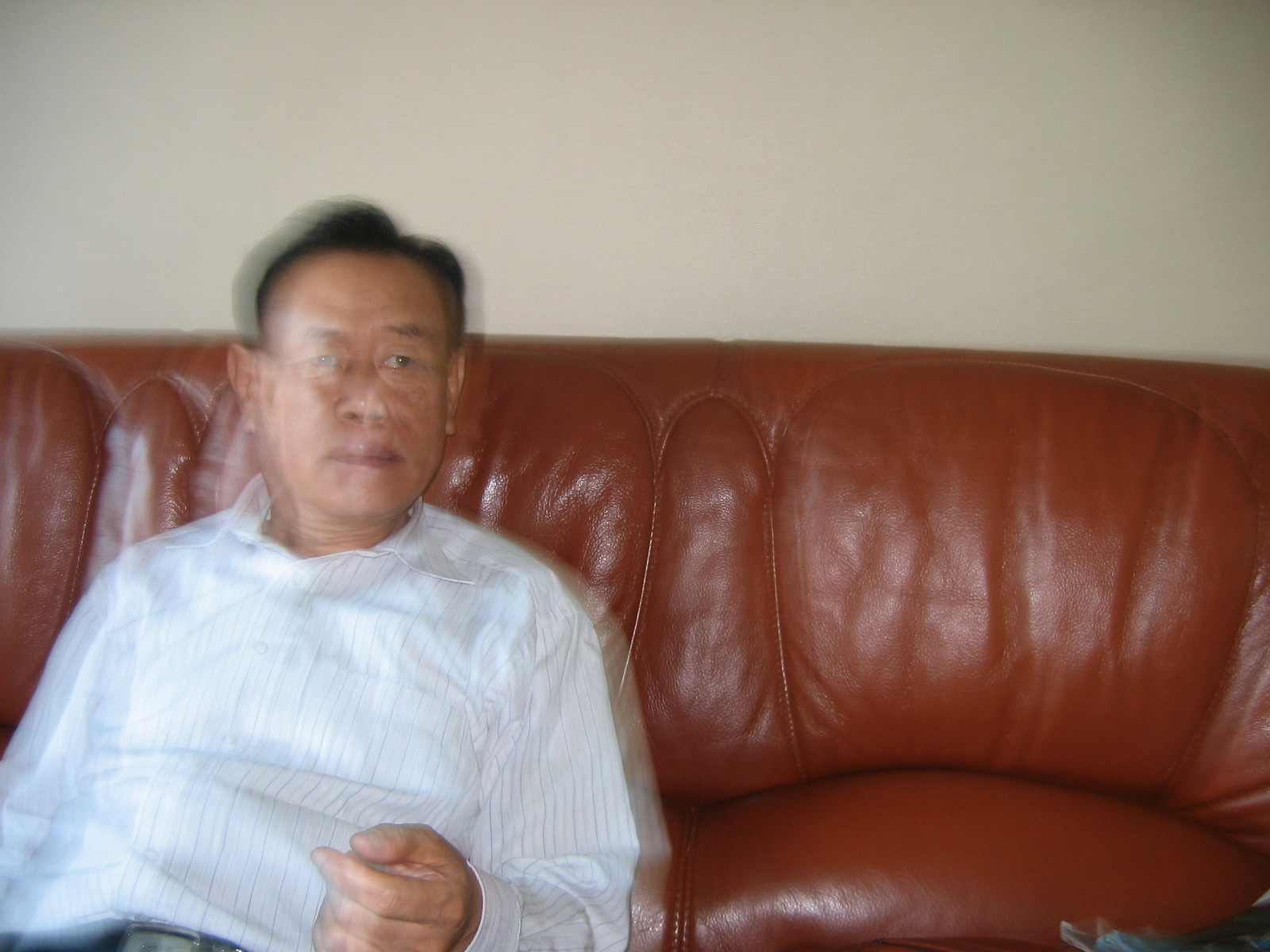The photograph features a blurred man with short black hair seated on the left side of a reddish-orange-brown or mahogany-colored leather couch, with noticeable stitching on the back cushion. He is positioned inside a residential-type home in front of a beige or off-white wall. The man's upper body is visible, dressed in a long-sleeved, white button-up shirt with subtle pinstripes that could be gray or blue. His right arm rests at his side, and his left arm is bent, extending forward with his hand slightly cupped, revealing his thumb and fingers. He appears to be looking off to the right side of the photograph, giving an impression of motion or recline. The image also captures a glimpse of the top of a silver belt buckle and the edge of black pants in the bottom left corner.